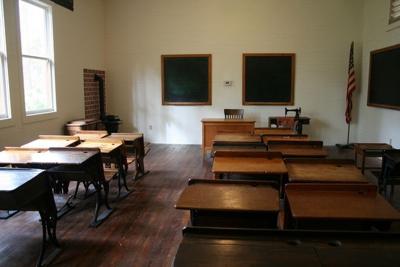This photograph showcases a vintage classroom with distinct antique features. The room is arranged with three rows of solid wooden desks, each row containing about three columns of lift-top desks with Victorian metal frames. At the head of the classroom stands a teacher's desk, beside which rests what seems to be an antique black metal sewing machine, possibly a Singer Featherweight model. The classroom is equipped with two medium-sized blackboards at the front and an additional blackboard on the right side. Positioned between the two front blackboards is a thermostat. An American flag occupies the right corner near the teacher's desk, adding a patriotic touch to the setting. The classroom's left side is lined with tall windows that allow ample sunlight to flood the room, highlighting the dated furnishings. In the left corner, there appears to be a brick wall with a stove, potentially a wood-burning or pot-bellied stove, with a pipe leading into the wall, contributing to the historical ambiance. The room, indicative of a bygone era, is a far cry from a modern school setting.